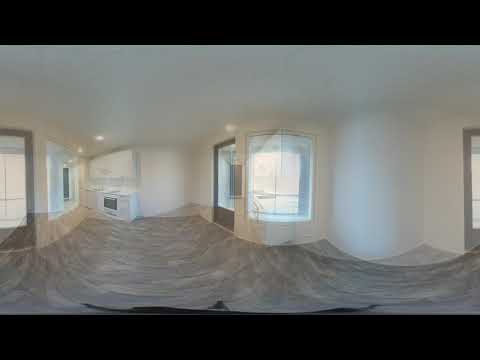The image depicts a vacant interior area of a house or apartment with distinct black borders at the top and bottom, giving it a framed appearance. The white walls and ceiling create a stark, clean setting. On the very right side of the image, a door is partially cut off by the edge. To the left, a semicircular wall feature juts out, followed by another protrusion housing a window with sunlight shining through. Farther in the background, multiple doorways are visible, suggesting access to different rooms. One of these doorways appears to lead to a kitchen area, identifiable by what seems to be a stove. The room in the foreground features a gray floor, described variably as being covered by a tarp or having a wavy, overlaid appearance, possibly due to photographic processing or stitching artifacts. The floor's texture includes light gray and white scribble-like patterns. The overall lighting is enhanced by some overhead lights. Despite the chaos due to the image overlay, the space remains clearly vacant, adding to its stark, uninhabited look.